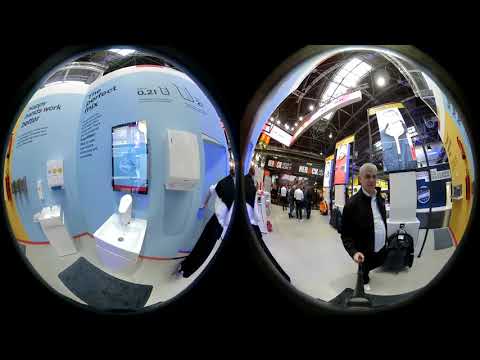In the image, two distorted, egg-shaped photographs reflect a 360 VR perspective, set against a solid black background. These two images sit directly next to each other, centered within the frame. On the left, a fisheye lens captures a detailed home improvement display, featuring a room with a carpet, a sink, and various wall-mounted items and writing. The scene, which appears slightly wavy due to the lens distortion, is likely part of a display at a convention hall or museum. On the right, another fisheye lens showcases a well-dressed man taking a selfie with a stick, under excellent indoor lighting, surrounded by posters and ceiling lights. The predominant colors in the scene include black, yellow, red, light blue, gray, dark blue, and orange. Despite the rich visual details, no text is readable anywhere in the image, reinforcing the visual focus on the vibrant convention or exhibit setting.